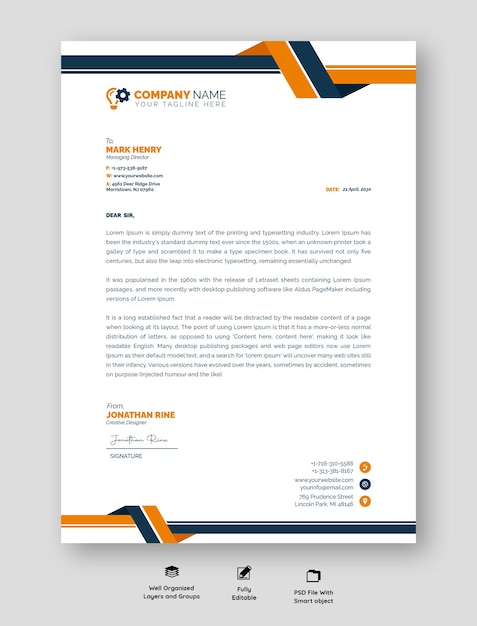This image showcases a detailed mock-up of a branded company letterhead template, intended as a display of a freelance designer's services. The letterhead features a white sheet with a prominent orange and blue knotted ribbon design at the top and bottom borders. At the upper-left corner, there is a placeholder for the company logo, depicted as an orange light bulb and a black settings wheel, and the editable text "company name, your tagline here."

The content of the letter begins with "Dear Sir," followed by several paragraphs of placeholder text in small print, demonstrating a typical layout for official company communications. The text includes the common "Lorem Ipsum" type, showcasing the layout as opposed to conveying actual information. On the top right, the date "23rd April 2013" is displayed, and at the bottom left, the letter is signed by "Jonathan Ryan, Creative Designer," with a space for an actual signature.

The image background is green, and interestingly, includes a set of icons at the bottom of the frame, each with accompanying details about the template's features: 
1. A stack of files with the caption "Well-organized layers and groups."
2. A pen indicating "Fully editable."
3. A folder labeled "PSD file with smart objects."

Additional placeholders are included for contact information, such as phone numbers, a website URL, an email, and a physical address, providing a comprehensive example of a professional letterhead layout. This mock-up is encased in a gray border, highlighting its role as a customizable template ready for client specifications.